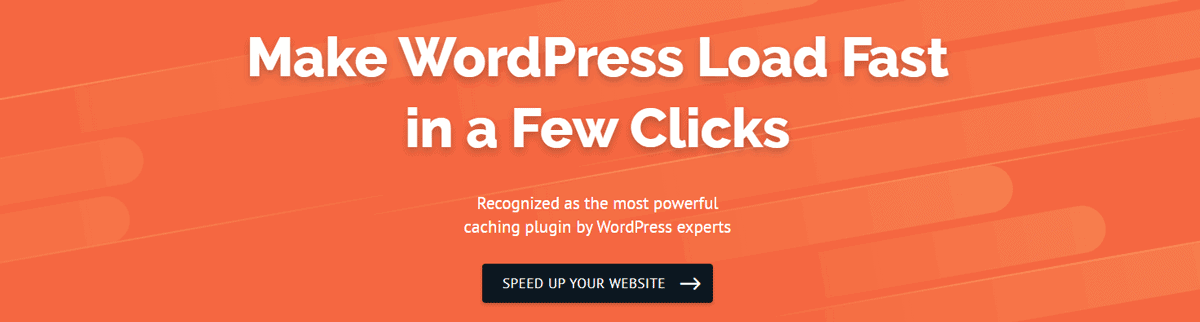This image is an advertisement designed for a desktop interface, as indicated by its large width and overall size. The background features a gradient of orange shades, composed of elongated rectangles with curved edges, resembling fingers pointing toward the center. These rectangles, numbering between seven and nine, create a dynamic backdrop.

Prominently centered in the image, there is a bold, white title in title case that reads, "Make WordPress Load Fast in a Few Clicks." Directly beneath it, in significantly smaller, white text, the centered alignment continues with the phrase: "Recognized as the Most Powerful Caching Plugin by WordPress Experts," emphasizing the plugin's credibility.

Below this text block is a black rectangle containing a call-to-action in white, all-caps lettering, which says "SPEED UP YOUR WEBSITE," accompanied by a right-pointing arrow. This element directs the viewer's attention towards further engagement. Overall, the image effectively promotes a WordPress plugin dedicated to enhancing website speed.